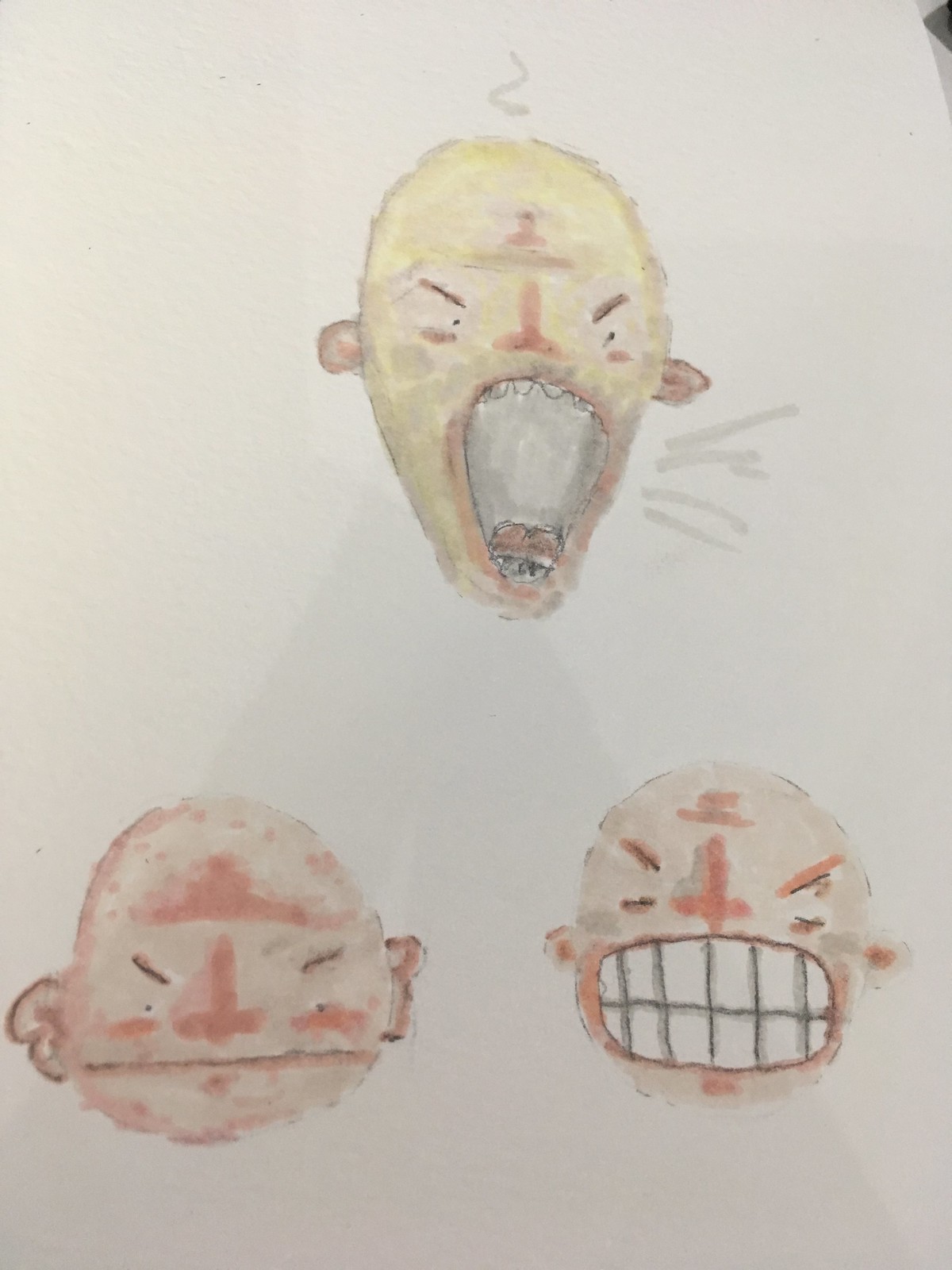The image features a white piece of paper, resembling a sketchbook, adorned with three expressive faces. The composition suggests an artistic style that begins with pencil sketches and is enhanced with watercolors. The primary face is located at the top center. This face is rendered with a predominantly yellowish hue and depicts a shouting expression, its mouth agape to reveal a gray-toned interior with visible tongue and upper teeth. The eyes are mere slits, and two ears are faintly visible, lending the face an almost Asian-inspired stylistic quality. Surrounding the primary colors of red and yellow, gray accents punctuate the dramatic emotion conveyed.

Below are two additional faces, maintaining the same color palette and stylistic elements. The face on the left exhibits a solemn demeanor, with closed eyes and a straight mouth, embodying a subdued expression. In contrast, the face on the right conveys intense anger, characterized by tightly clenched, prominent teeth and the same grayish complexion interspersed with red markings. These varied expressions collectively create a vivid display of human emotion through a minimalist yet powerful artistic lens.